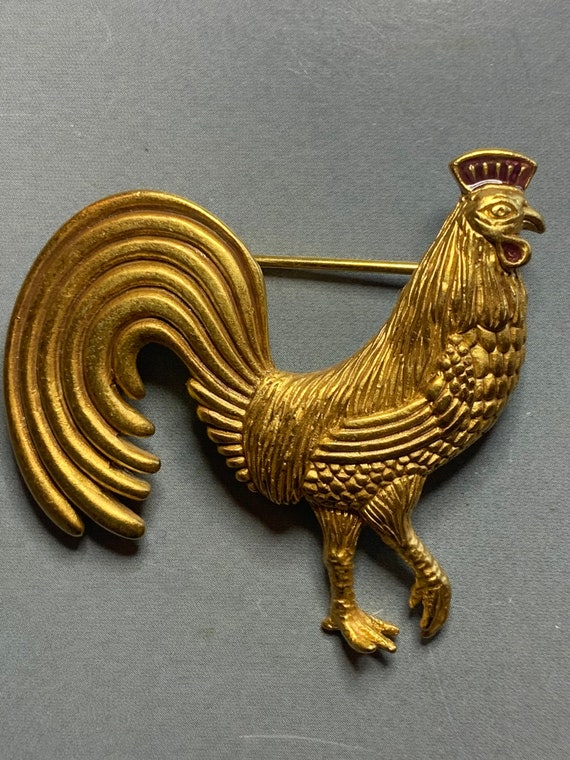This image showcases a detailed, vintage gold pin or brooch in the shape of a rooster, set against a simple gray background that makes the gold really pop. The gold rooster, likely an antique, is intricately designed with extensive etching that highlights the ornate feathers. The feathers vary in length, with the longer ones forming a curved "C" shape for the tail. The rooster's head is held high, displaying its large gold comb and small beak, while it's depicted in a walking stance with one leg lifted, giving a sense of movement. Its long neck, elaborate plumage, and the visible pin bar on the back indicate it's made for fastening to clothing, showcasing its craftsmanship and vintage charm.